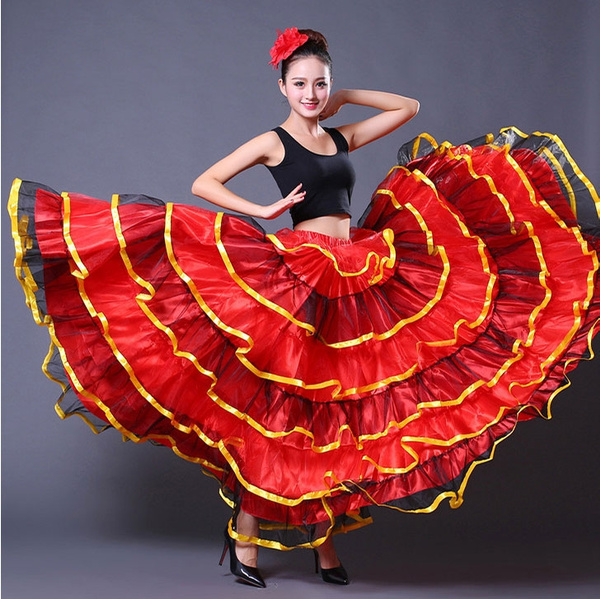The large square image features a young woman, likely in her late teens or early 20s, standing in the center against a solid gray backdrop that darkens on the lower right due to her shadow. She has light skin and is dressed in a vibrant and elaborate outfit reminiscent of a Spanish dancer or flamenco performer. Her hair is pulled up into a big bun adorned with a large red hibiscus flower, and she wears dark pink lipstick.

Her attire includes a black crop top that exposes her midriff and a voluminous, eye-catching red dress with layers of ruffled fabric. The dress is intricately detailed, with approximately five layers of ruffles, each trimmed with yellow ribbon—some of which are hanging loosely. Her left leg is positioned forward and slightly to the side, giving a sense of movement as if she might be dancing or twisting. 

Her right arm is bent with her hand resting on her waist, while her left arm is also bent with her hand positioned behind her neck. Her bare feet are visible, adorned with black high heels. She is smiling directly at the camera, capturing a moment full of grace and poise, as her flowing dress spreads out dramatically around her, creating an arc that almost touches the ground near her ankles, signifying a possible dynamic motion.

The background appears to be a continuous piece of fabric, giving a soft, mixed gray appearance that complements the vivid colors of her attire. The overall composition highlights her energetic and joyful presence, emphasizing the dance-like elegance encapsulated in this portrait.